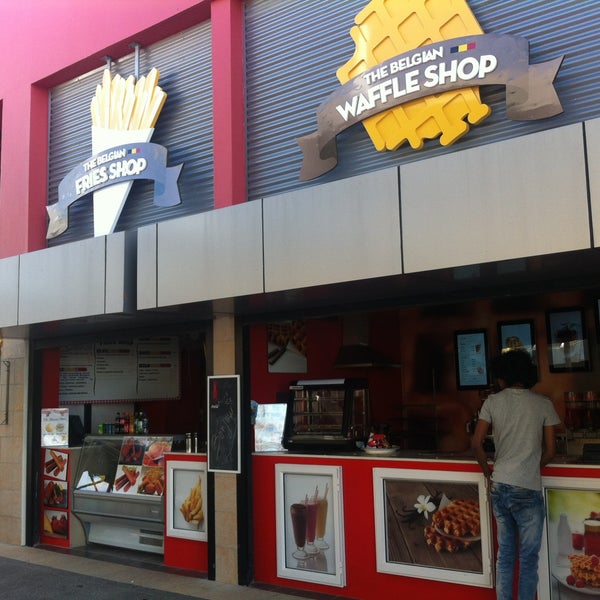This image captures a quaint, likely outdoor shopping center featuring two closely situated food shops. On the left, slightly set back, stands the Belgian Fry Shop, characterized by a prominent sign displaying a large sack of fries. The shop’s facade also includes pictures of French fries or Belgian fries, with a detailed menu visible in the background. To the right and more towards the foreground is the Belgian Waffle Shop. A single customer, with his back turned to the camera, stands in front of this shop. Surrounding the front desk are images of Belgian waffles and milkshakes, along with a small heat container. Despite the dim lighting and relatively empty atmosphere, the shops vividly advertise a range of Belgian-themed delicacies, including waffles, milkshakes, fries, and possibly other items like mozzarella sticks and various breads.